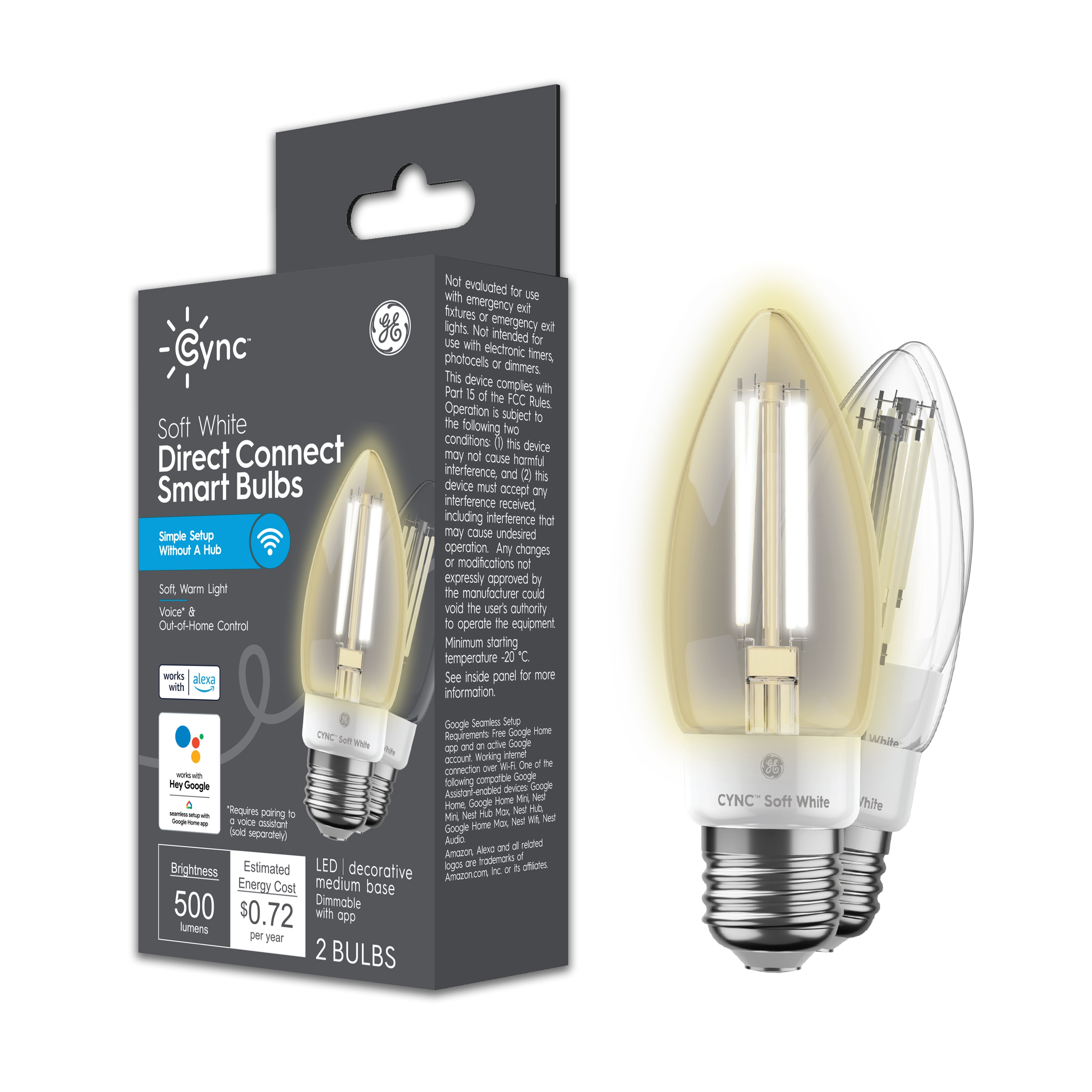The advertisement showcases SYNC Soft White Direct Connect Smart Bulbs by General Electric. On the left side, there's a light gray box featuring two flame-shaped, pyramid-like bulbs. The box prominently displays the GE logo in the top right corner and announces the product as a Direct Connect Smart Bulb, requiring no hub for setup, as highlighted by a blue banner with a Wi-Fi signal icon. Below, it includes compatibility icons for Alexa and Google Assistant. The box also details the brightness at 500 lumens and the estimated energy cost of $0.72 per year. On the right side of the ad, two enlarged images of the bulbs show the front bulb lit and the back bulb unlit, each marked with the SYNC branding and "soft white." Additional text on the box mentions features such as Voice and Out of Home Control and Soft Warm Light.